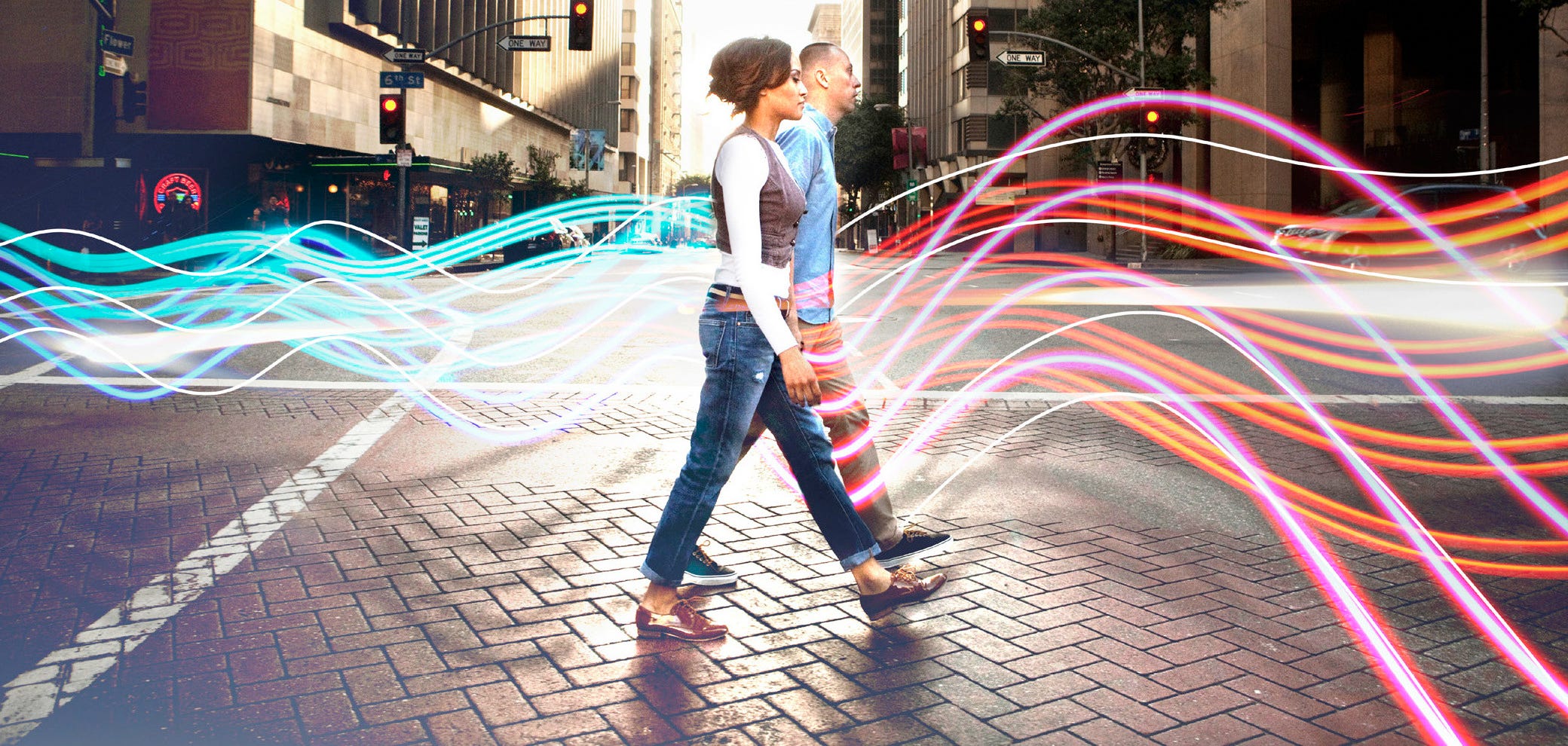A horizontally-oriented photograph with some digital editing captures a bustling urban scene featuring two pedestrians crossing a wide brick road in the middle of a city. Tall buildings flank both sides of the street, and the surroundings include various store signs, logos, and a noticeable stoplight with all lights red. The road is composed of primarily red or dark grey bricks, neatly lined with a white traffic stripe on the left. Both individuals, appearing to be in their 20s or 30s with light brown skin, are walking towards the right side of the image. The woman, closer to the foreground, is dressed in blue jeans, brown shoes, a white long-sleeved shirt, and a grey vest. The man, slightly behind her, sports a blue button-down shirt, dark pants, and black and white shoes. Their side profiles are clearly visible as they move forward. Enhancing the visual interest, digital neon-colored waves—consisting of blue, pink, orange, and white hues—trace their movement across the scene, adding a surreal touch to the realistic urban backdrop.